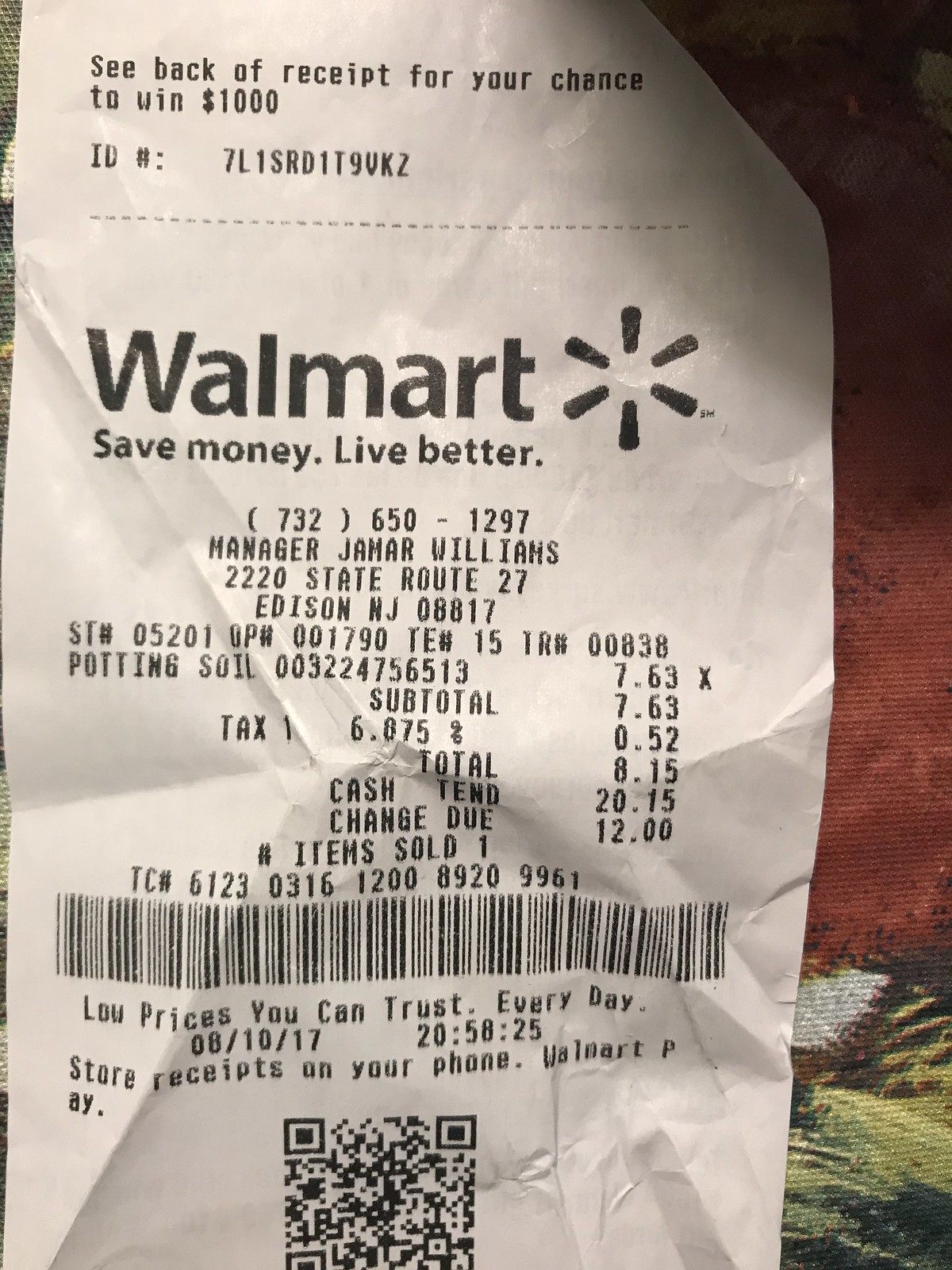This close-up image features a crumpled Walmart receipt positioned to the left. The top of the receipt advertises a chance to win $1,000 with an ID number displayed beneath this message. Directly below, the Walmart logo appears alongside the slogan "Save Money, Live Better." The manager, Jemar Williams, and the location, Edison, New Jersey, are printed, followed by the purchase details. The receipt shows two items of potting soil, each priced at $7.63, with a subtotal including a 52-cent tax, summing to $20.15. A barcode and messages of "Low Prices You Can Trust Every Day" promote Walmart’s value proposition. The transaction occurred on August 10, 2017, at 20:58:25. Additionally, the background to the right features part of a folded fabric with an orange top transitioning into green and white sections.